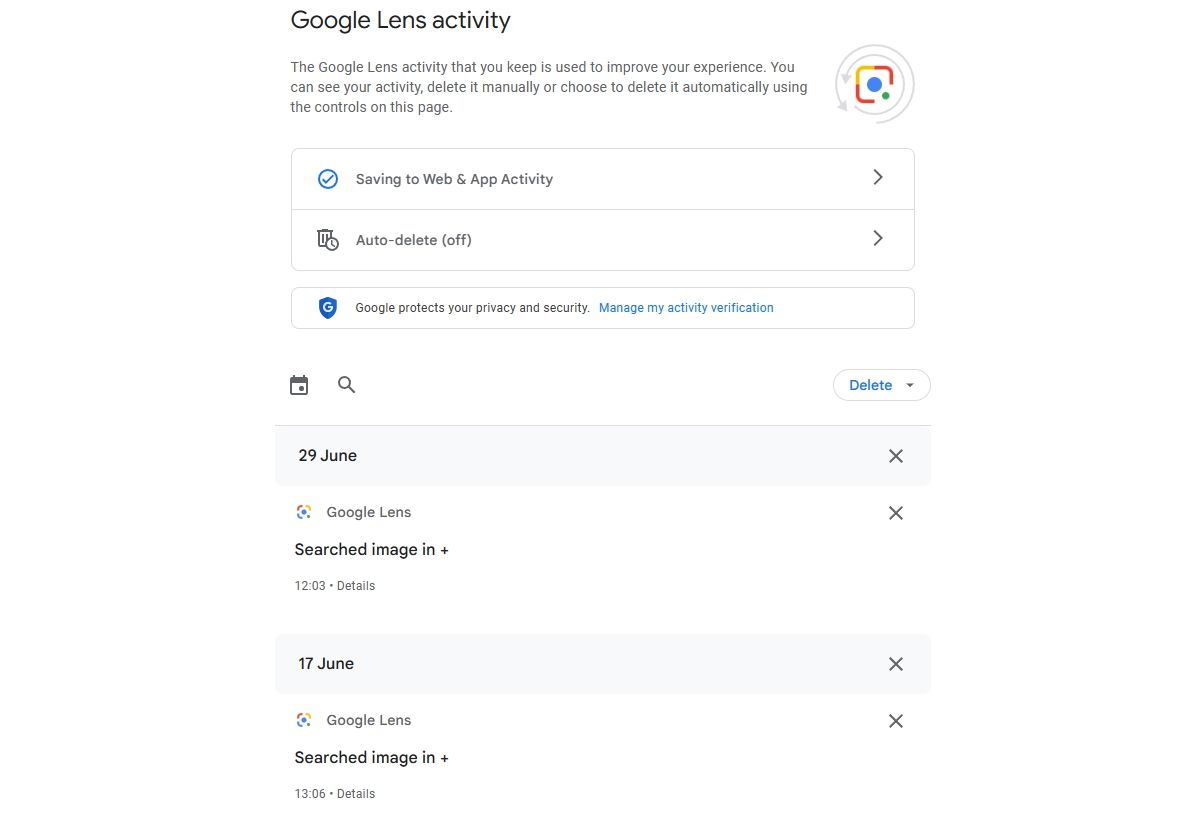The screenshot from the website showcases the "Google Lens Activity" page. At the top, the heading "Google Lens Activity" is displayed in black print with the 'G' and 'L' capitalized. Beneath this heading, a message conveys that the Google Lens Activity retained on the page is utilized to enhance user experience. Users are informed that they can review, manually delete, or set up automatic deletion of their activity using the controls provided on the page.

Further down, there is a section featuring a blue circular icon with a white check mark inside, accompanied by the text "Saving to Web & App Activity." Adjacent to this section is a right-facing arrow. Below, a trash can icon with a small clock symbol overlaid on it signifies that the auto-delete feature is turned off, with another right-facing arrow next to it.

A shield icon with a 'G' inside follows, paired with a message in blue text stating, "Google protects your privacy and security," along with a "Manage my activity verification" link in blue.

Subsequently, a calendar and magnifying glass icon appear, indicating specific search dates and times. Dates listed include "29 June" with "Google Lens searched image" at 12:03, and "17 June" with "Google Lens searched image" at 13:06, each followed by the word "details."

To the right side of each entry is an 'X' button that allows users to delete individual items. Above these 'X' buttons, a small oval button with the text "Delete" in blue provides a dropdown menu option for bulk deletion.